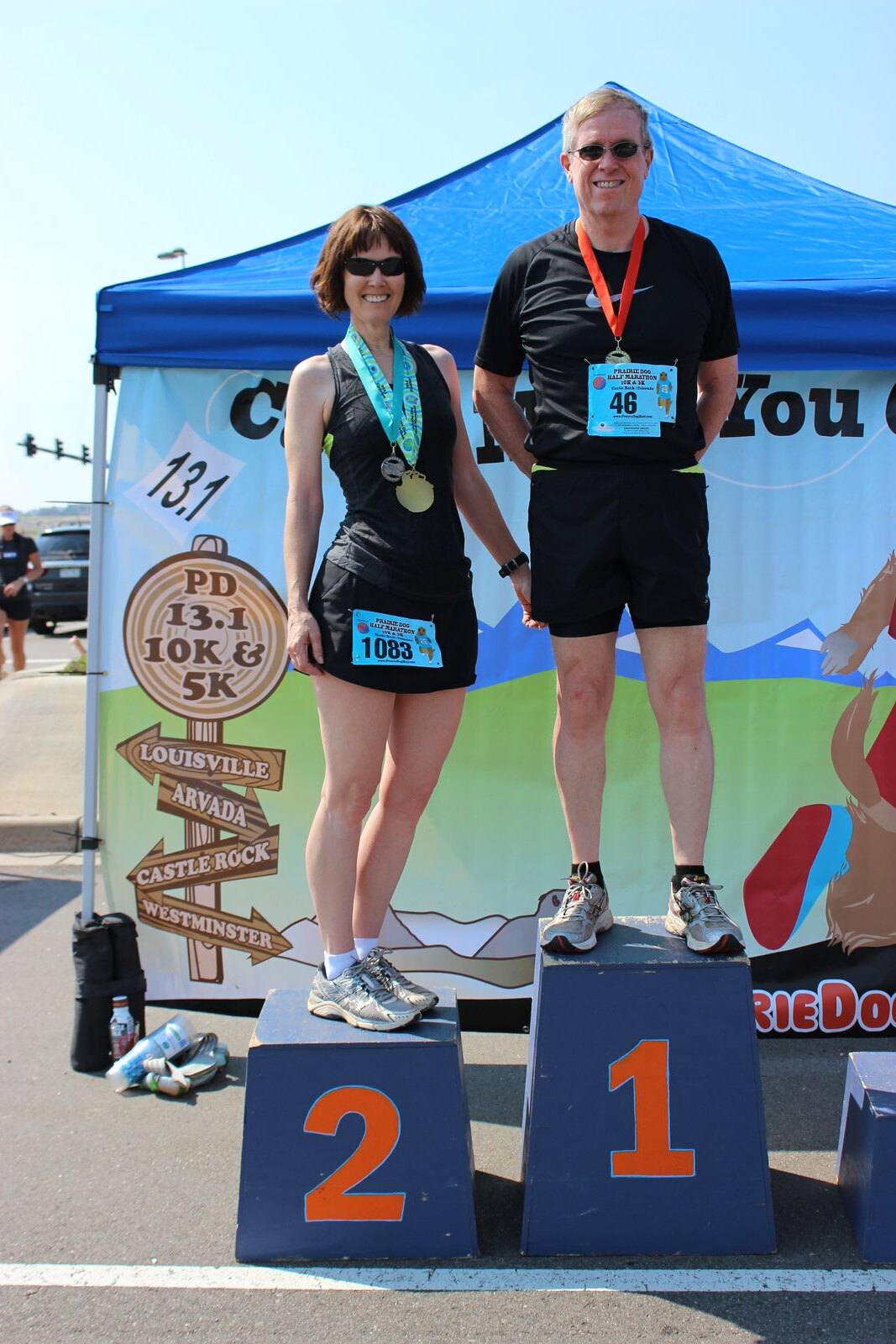A vibrant, sunny day provides the perfect backdrop for a photograph taken after an athletic event in an open field. In the center of the image, a three-tier podium displays the numbers one, two, and three in bold orange. Atop the highest platform, marked "1", stands a tall white man sporting short blonde hair, dark sunglasses, and an orange lanyard with a card displaying the number 46. He wears a black Nike running shirt, black shorts, and sneakers. Beside him, on the number "2" podium, a white woman with short brown hair smiles brightly, donning black sunglasses, a black running top, black shorts, and sneakers. Around her neck are two medals hanging from blue lanyards, and her running number label, "1083," is pinned to her shorts.

Behind the podium, a blue-topped tent features partially obscured signage, including partial text like "Louisville" and "Castle Rock," and illustrative signposts indicating distances like PD 13.1, 10K, and 5K, with directional arrows pointing to various locations. To the left of the frame, a man stands near a police SUV, visible alongside three traffic lights. The predominant colors in the scene are blue, green, white, and orange, emphasizing the celebratory nature of the day.